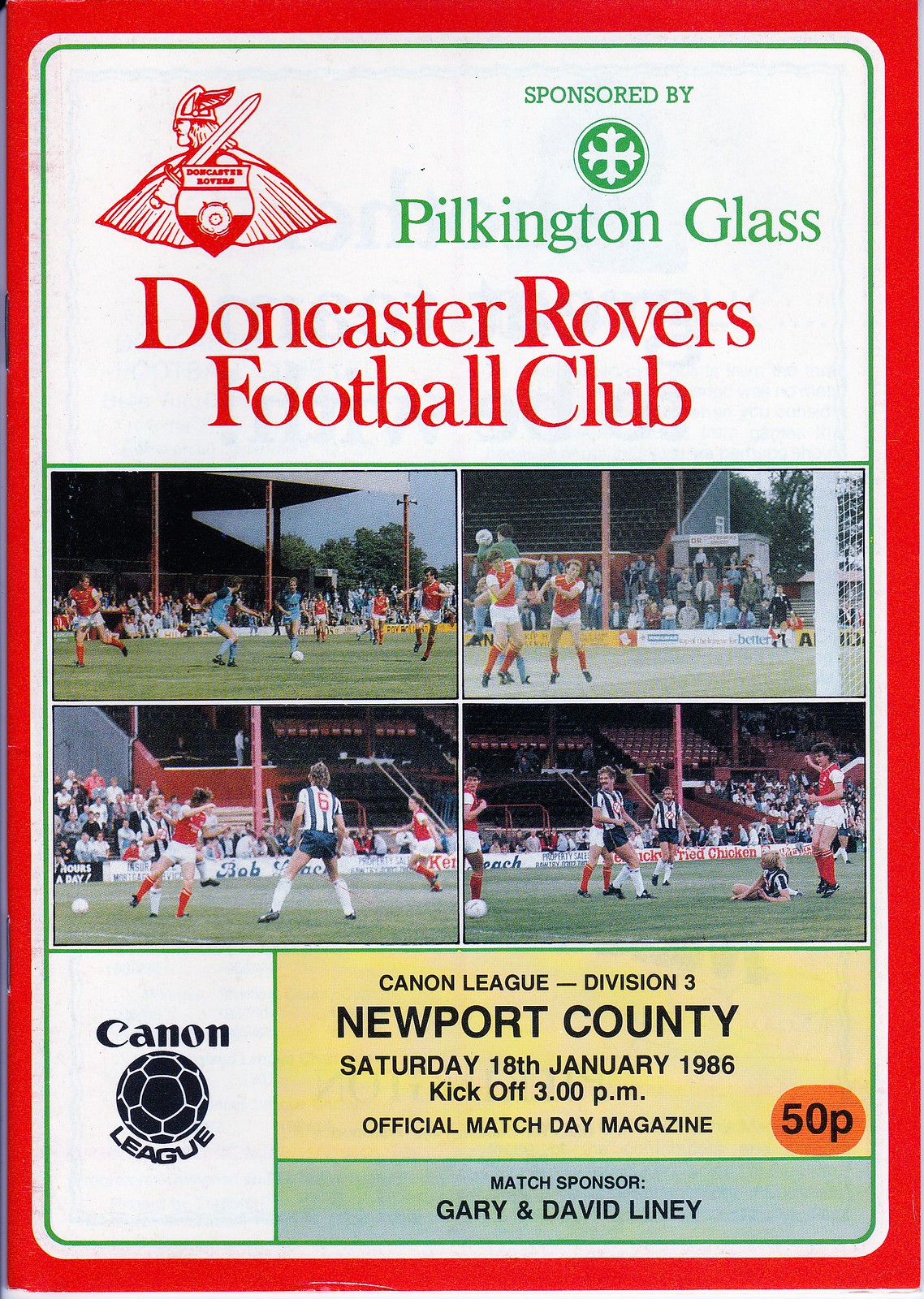The brochure features a distinct red outline with an inner green border. At the top, there's a prominent red illustration of a Viking holding a sword with a shield and a Viking hat adorned with wings. Adjacent to this Viking image, in green text, is the caption "Sponsored by Pilkington Glass." Below, in striking red letters, the brochure declares "Doncaster Rovers Football Club." Underneath, three photographs display various football games, featuring players in red, blue, and striped uniforms, with one player marked by a number six on the back of his jersey. The spectator stands appear sparsely populated, with more fans visible in the lower sections. At the bottom of the brochure, a soccer ball icon houses the text "Cannon League Division Three," in reference to the match: Newport County, Saturday, 18th of January 1986, kickoff at 3 p.m. Additionally, it marks this as the "official Match Day magazine," with Gary and David Linney listed as match sponsors. A noticeable orange circle with "50P" in black letters also stands out against the colorful and detailed design of the brochure.